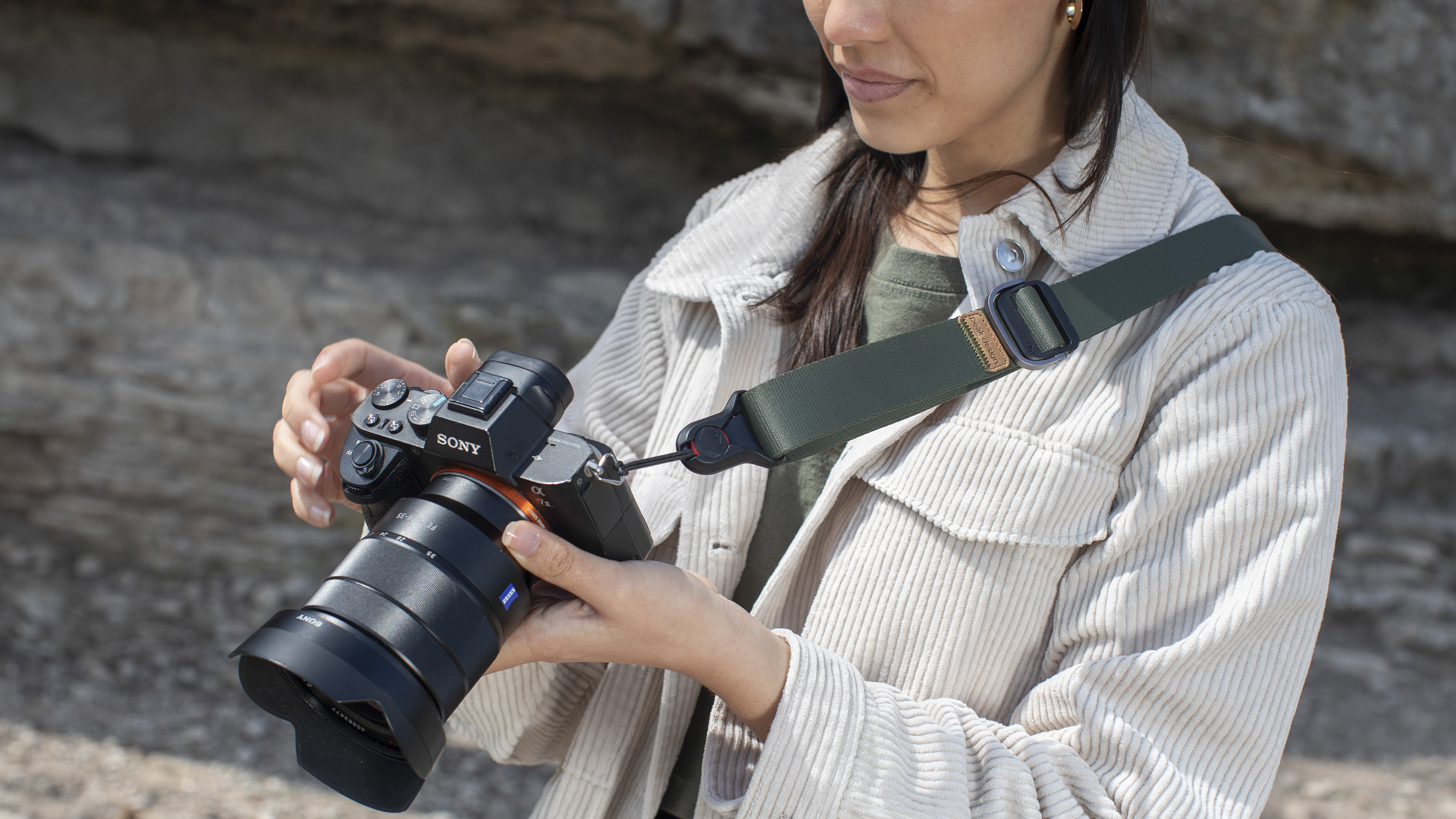In this detailed color photograph, we see a woman in her early 30s standing on the right side of the image, gazing down at a black Sony camera with a long zoom lens extended towards the bottom left. Cropped from mid-nose to mid-chest, she has long, dark hair and is wearing a light brown corduroy jacket over an olive green t-shirt. The camera is suspended from a wide black strap with a buckle, draped over her left shoulder to the bottom left of the image. Partially visible is an earring in her ear. The background features an out-of-focus rocky surface in shades of gray and brown, adding a subtle textured backdrop to the scene. The photograph is in landscape orientation and follows a representational realism style.